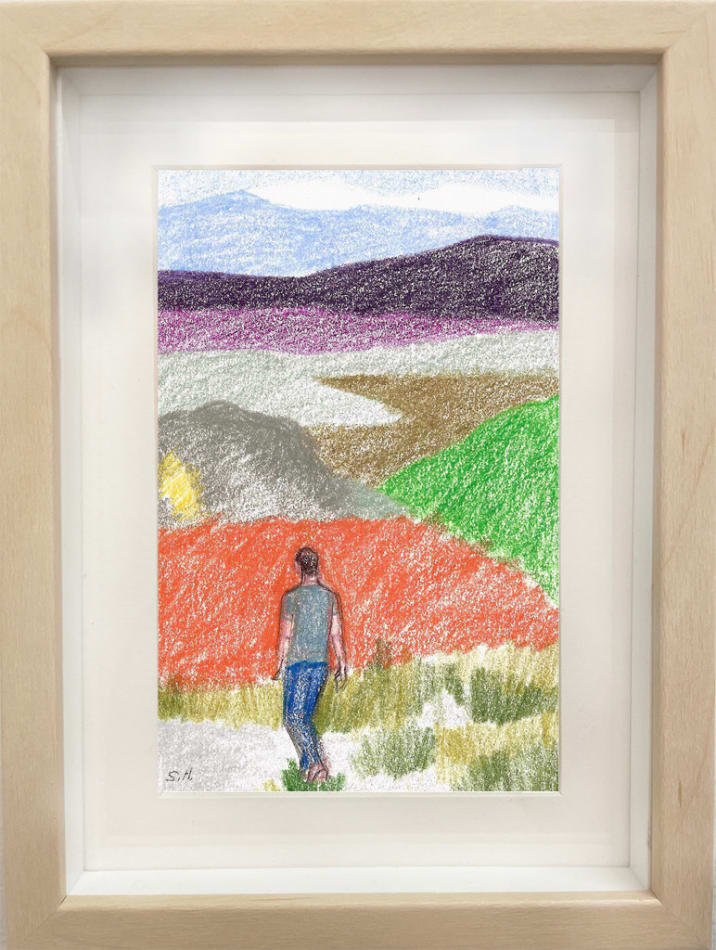This image features a photograph of a painting, displayed indoors against a wall. The painting, encased in a light brown frame with white matting, is drawn in a crayon-like style and depicts an expansive outdoor landscape. The scene captures a man, wearing a green short-sleeved shirt, blue jeans, and brown shoes, facing away from the viewer and walking along a pathway. The pathway consists of white sand, green grass, and varying flatlands that blend in with a multi-colored field in the background. The vivid landscape features layers of color: yellow, green, and gray hills, transitioning to a purple field, culminating in distant gray and blue mountains beneath a blue sky. The lower left corner of the painting holds a signature "S a".